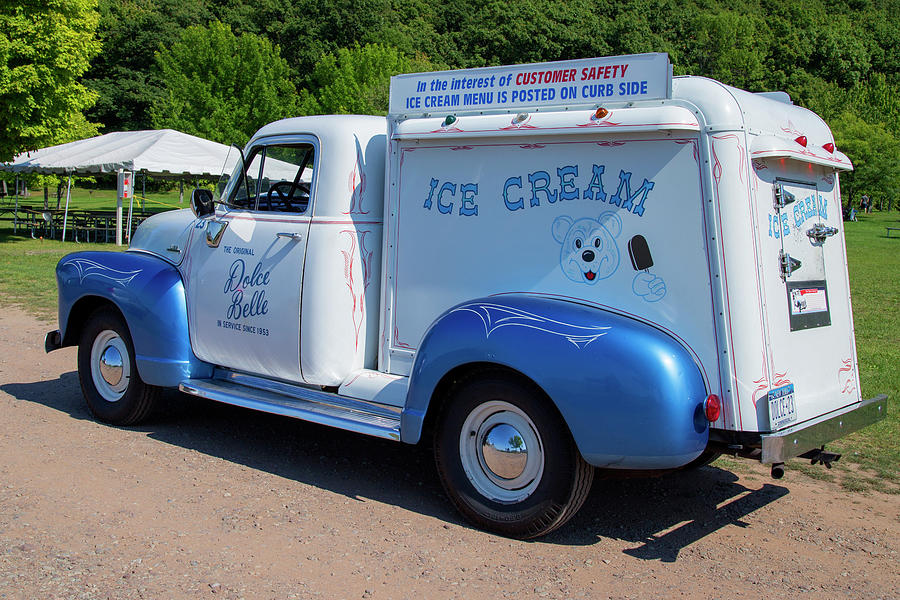This is a photograph of a vintage ice cream truck, reminiscent of the 60s or 70s, with a charmingly old-fashioned design. The truck itself is primarily white with light blue bumpers and fenders, and it features large, thick wheels with silver semicircles in the middle. A New York license plate on the back reads "Dolce 23." Prominent blue block lettering on the side and the back hatch spells out "ice cream," beneath which a friendly, smiling bear holding a chocolate ice cream popsicle is illustrated. Above this, a sign reads: "In the interest of customer safety, ice cream menu is posted on curbside." The front of the truck is adorned with the text "Dolce Belle, the original" and "In service since 1953" (erroneously noted as 1850 in one caption). The backdrop of the image showcases a beautiful, lush green forest with tall trees, and a tent with a white canopy is visible on the left. The truck is parked on a reddish dirt road scattered with stones, and patches of green grass peek through in the distance.